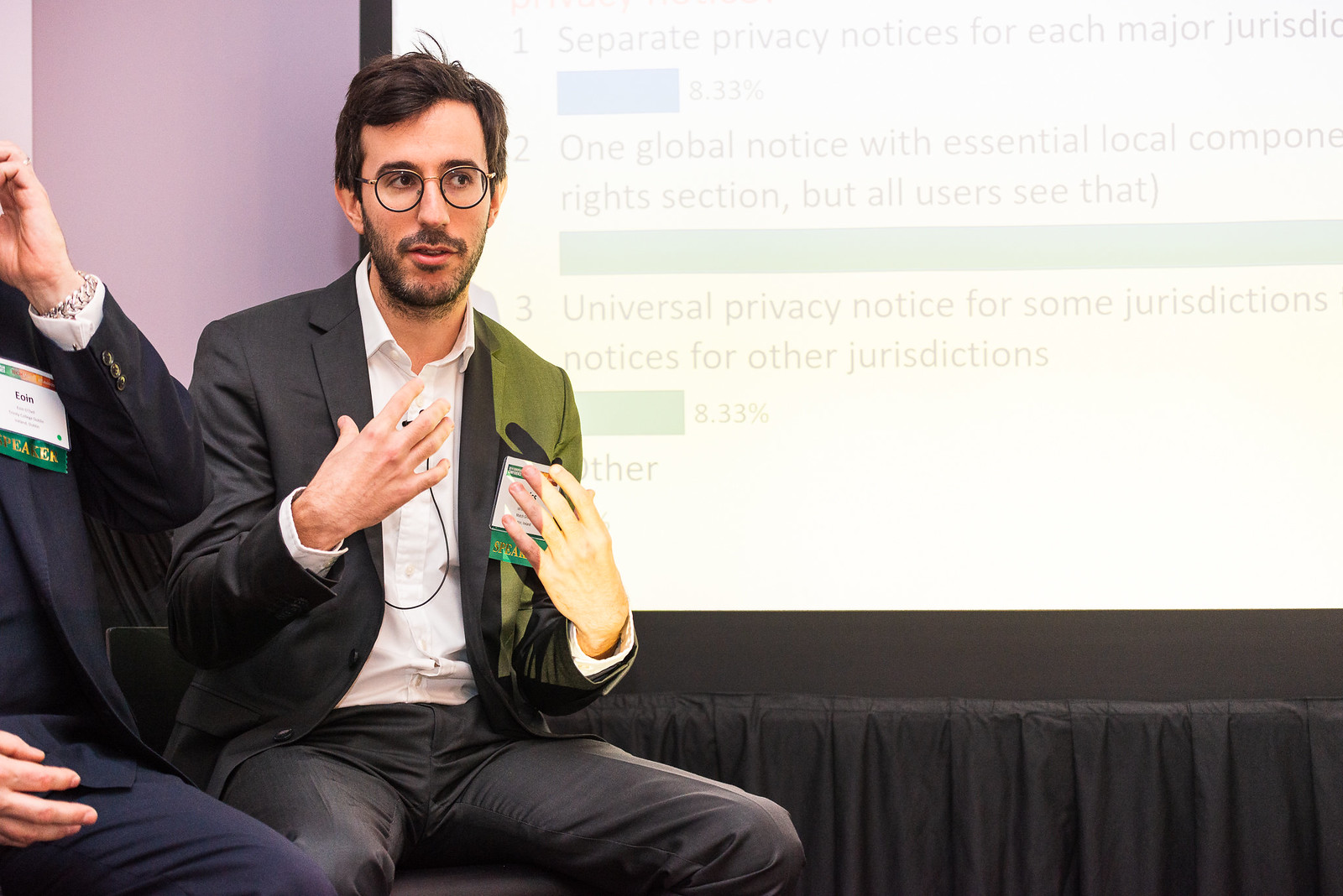This photograph captures a young man with dark brown hair, a short beard, and a mustache, speaking animatedly while seated at a conference. He's dressed in a white open-collared button-down shirt, a dark gray suit coat, and matching pants. A microphone is clipped to his shirt, and he wears eyeglasses, along with a name tag featuring multiple ribbons, suggesting his participation in a professional event, likely a learning conference. He is positioned to the left of another partially visible individual in a blue sport coat, also wearing various name tags. Both men appear to be on a stage, seated at a table covered with a black drape, typical of those used in conference rooms. Behind him, a screen projects several data graphs, including a notable blue bar indicating "8.3%" and a large green bar among other textual information related to privacy notices for different jurisdictions. The man's gestures and his engaged demeanor signify his active role in presenting the information to an audience.